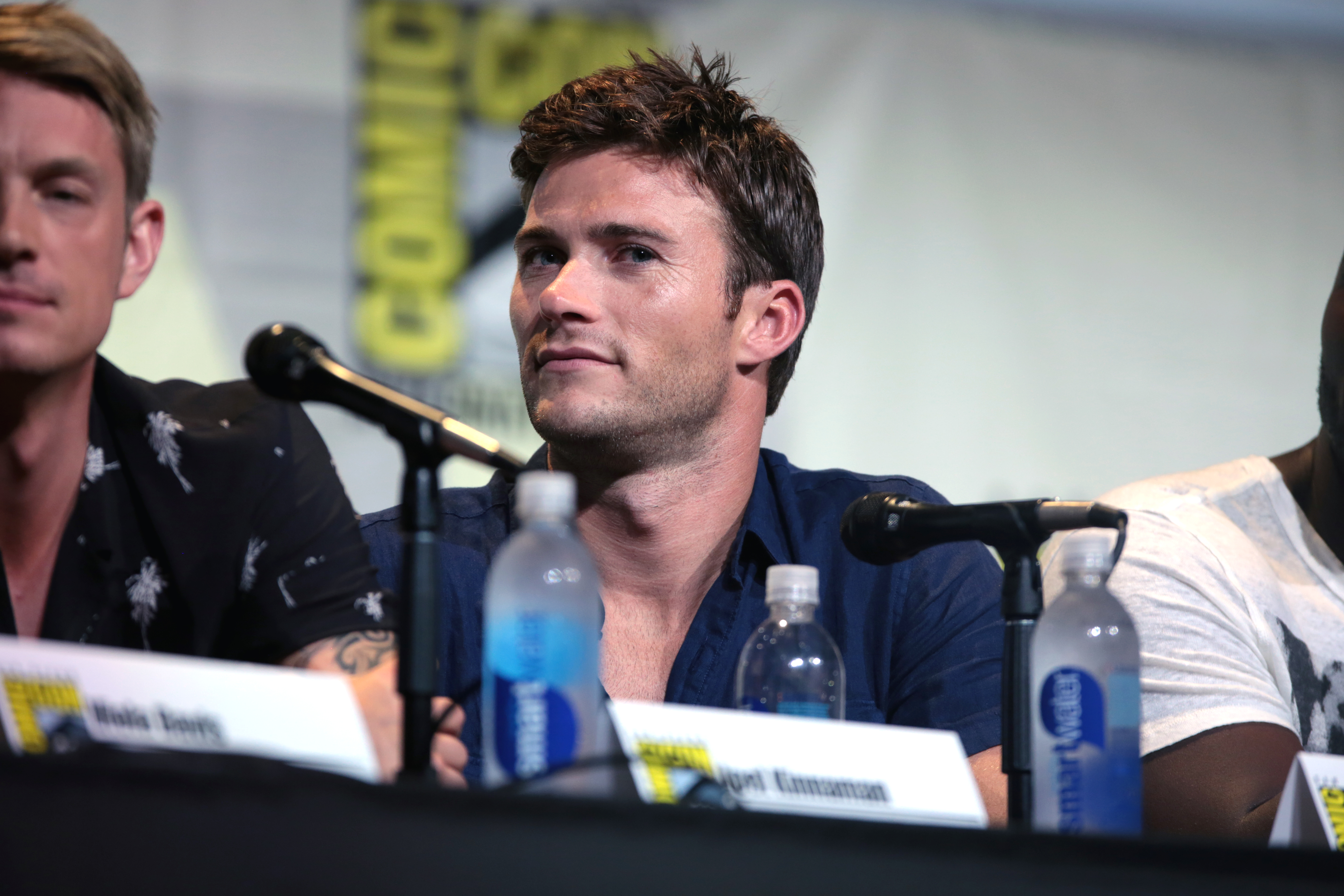The image captures a panel at a convention, potentially Comic-Con. Seated at a lengthy table are three men, with the focus primarily on the man in the center. This individual, who has short, dark hair and is wearing an open-collar, light dark blue short-sleeve shirt, appears to be glancing sidelong at the audience. To his left, only partially visible, is an African American man wearing a white t-shirt. His facial features are not discernible due to the angle. On the far left and minimally visible, a man with short blonde hair, a black t-shirt, and a tattoo on his left arm is seated. In front of each individual are bottles of Smartwater and placards that are too blurry to read. Positioned on the table are two microphones situated in front of the man in the blue shirt and the man in the black t-shirt. They sit against a backdrop featuring a white banner with partially obscured vertical yellow lettering, hinting at the possible word "COMIC."